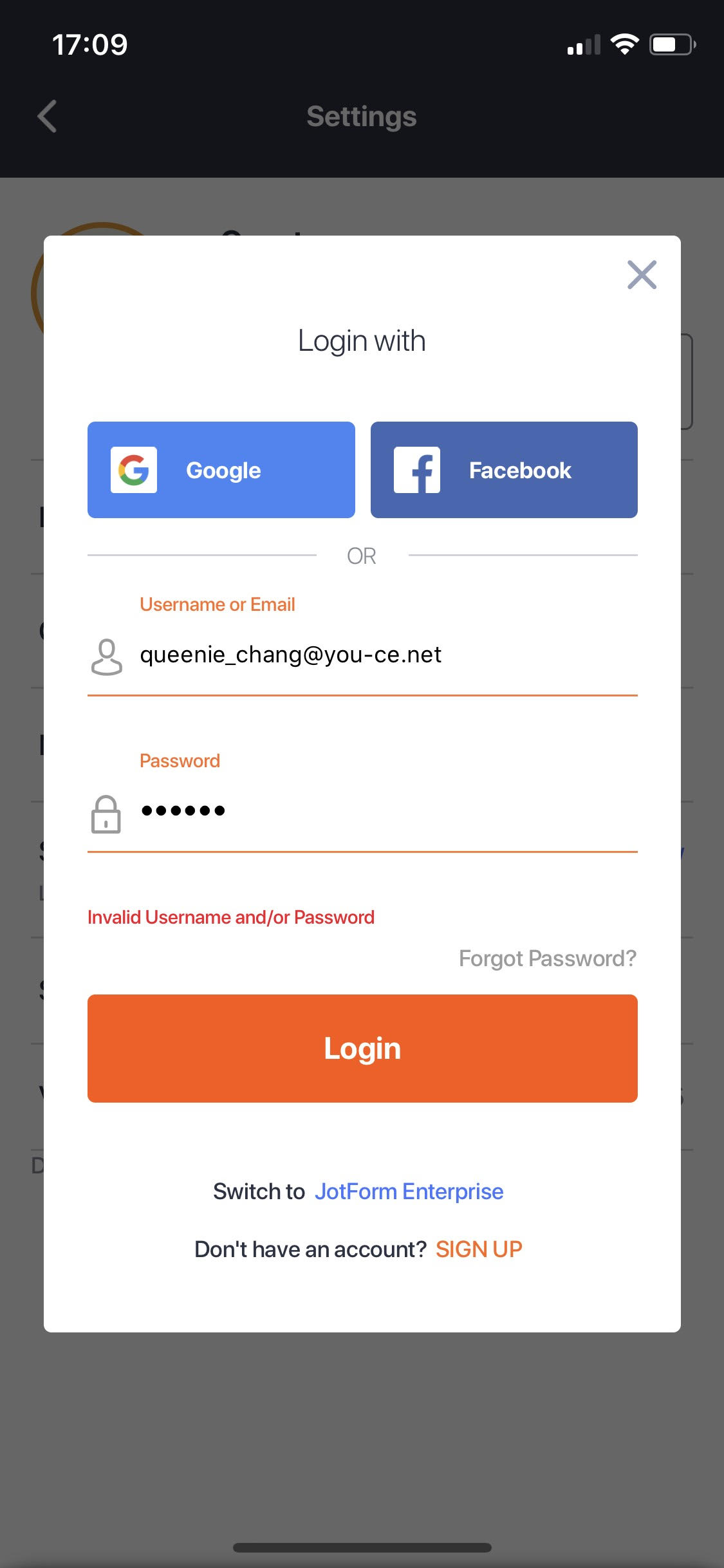This screenshot captures a mobile phone screen displaying a settings interface at 5:09 PM (1709 in military time). The upper left corner indicates two bars of internet connectivity, and the battery indicator shows slightly over 50% charge. A black bar spans the top, while the majority of the screen is occupied by an off-white pop-up window.

The pop-up window features a gray 'X' in the upper right corner for dismissal. Centered at the top is a small, dark gray text reading "Login With." Below this, there are two prominent buttons: one on the left labeled "Google" with its corresponding icon, and one on the right labeled "Facebook," also with its icon. Between these buttons is the word "OR" in uppercase, flanked on either side by horizontal lines.

Further down, in red text, is the prompt "Username or Email," adjacent to an icon resembling a person. The entered text here is "Queenie.change@" followed by placeholder text. Below this, another red prompt reads "Password," accompanied by a lock icon. The filled password triggers an error message in red text that reads "Invalid username and/or password." To address this, a clickable "Forgot Password" link is presented in gray text below the error message. At the bottom of the pop-up is an orange "Login" button, which remains unclickable due to the incorrect login details.